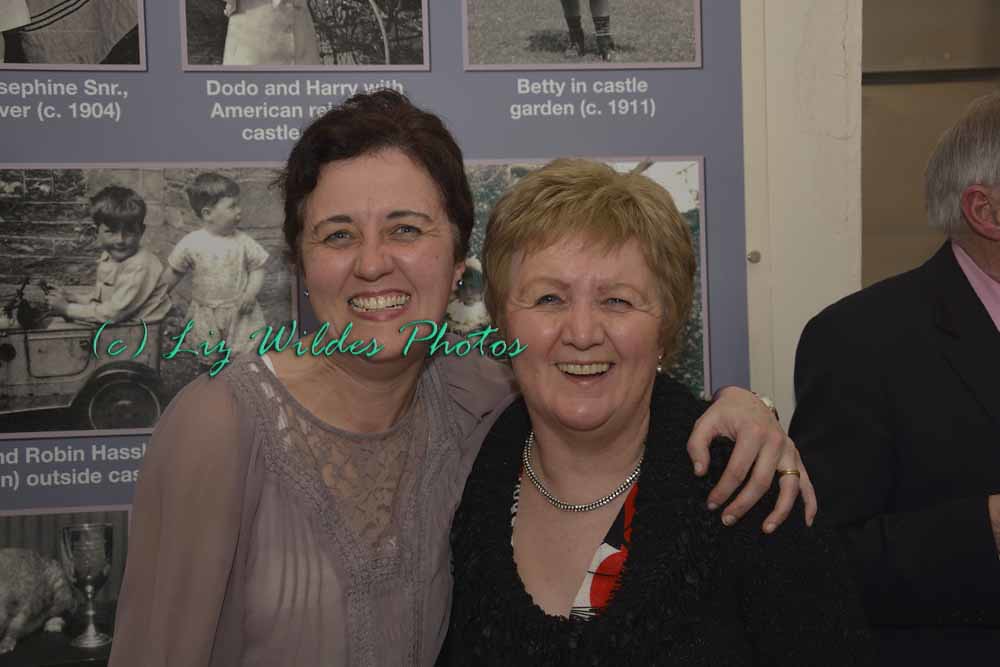In this photograph, two elderly women are smiling and posing together in front of a museum exhibit. The slightly taller woman on the left has her arm around the shorter woman on the right. She has fair skin and short dark brown hair, and she is beaming in a white tank top layered with a lace-detail purple long-sleeve shirt. The shorter woman has short blonde hair and fair skin, wearing a black, white, and red shirt underneath a black sweater, accessorized with a silver necklace. Behind them is a large purple sign adorned with black and white vintage photographs with captions. Immediately above the blonde woman, one caption reads, “Betty in Castle Garden circa 1911.” To their right, partially obscured, is the shoulder of an elderly man in a pink shirt and black suit, with gray hair.